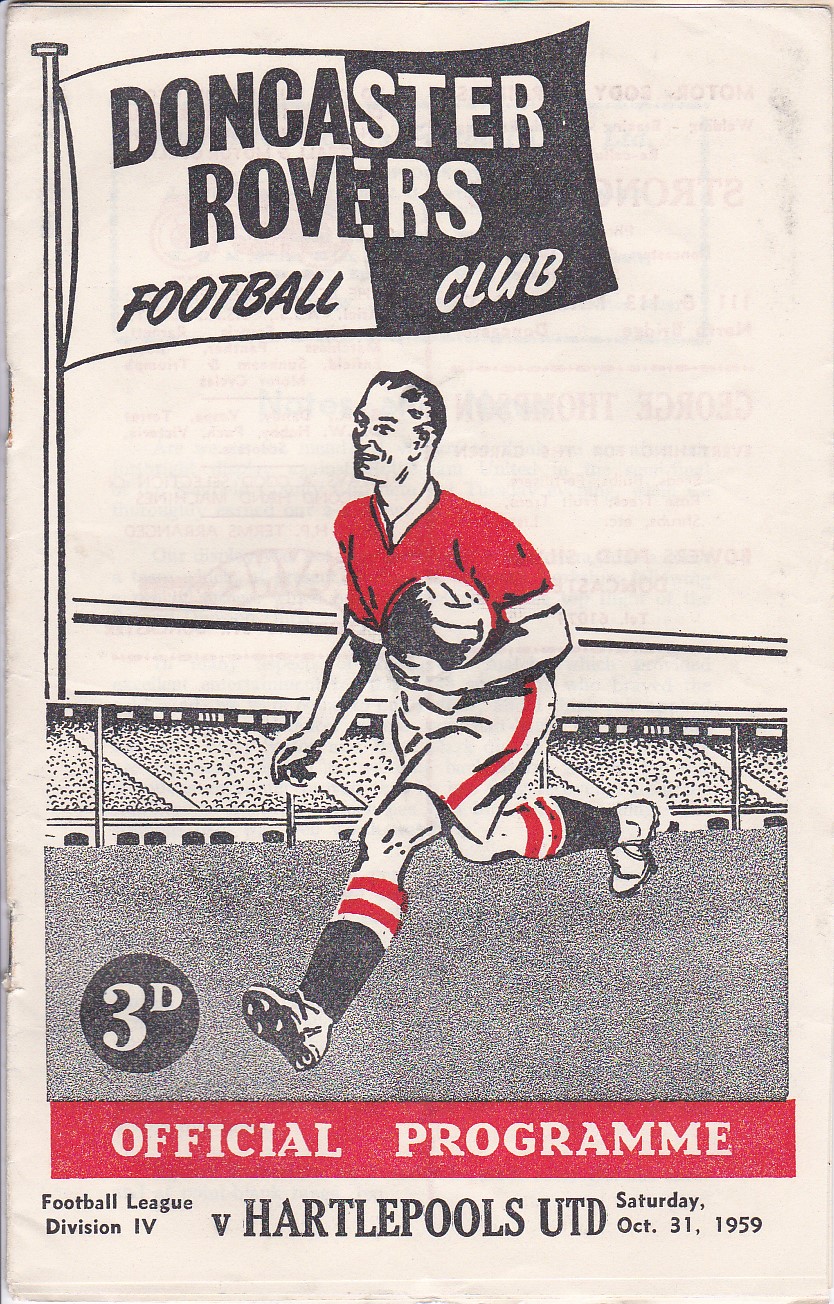The image is the cover of an old and slightly worn soccer program from October 31st, 1959. The main illustration, rendered in black, white, and red, depicts a soccer player in a red short-sleeved shirt running on the field, oddly holding a soccer ball in his hand. Behind him, the stands are filled with fans, indicated by tiny dots, creating a bustling background. In the upper left corner, an unfurled flag displays "Doncaster Rovers Football Club." In the bottom left corner, "3D" is marked inside a black circle. Beneath the illustration, a red horizontal stripe announces "Official Program," and in smaller black font below, it reads, "Football League Division IV versus Hartlepool's UTD, Saturday, October 31st, 1959."